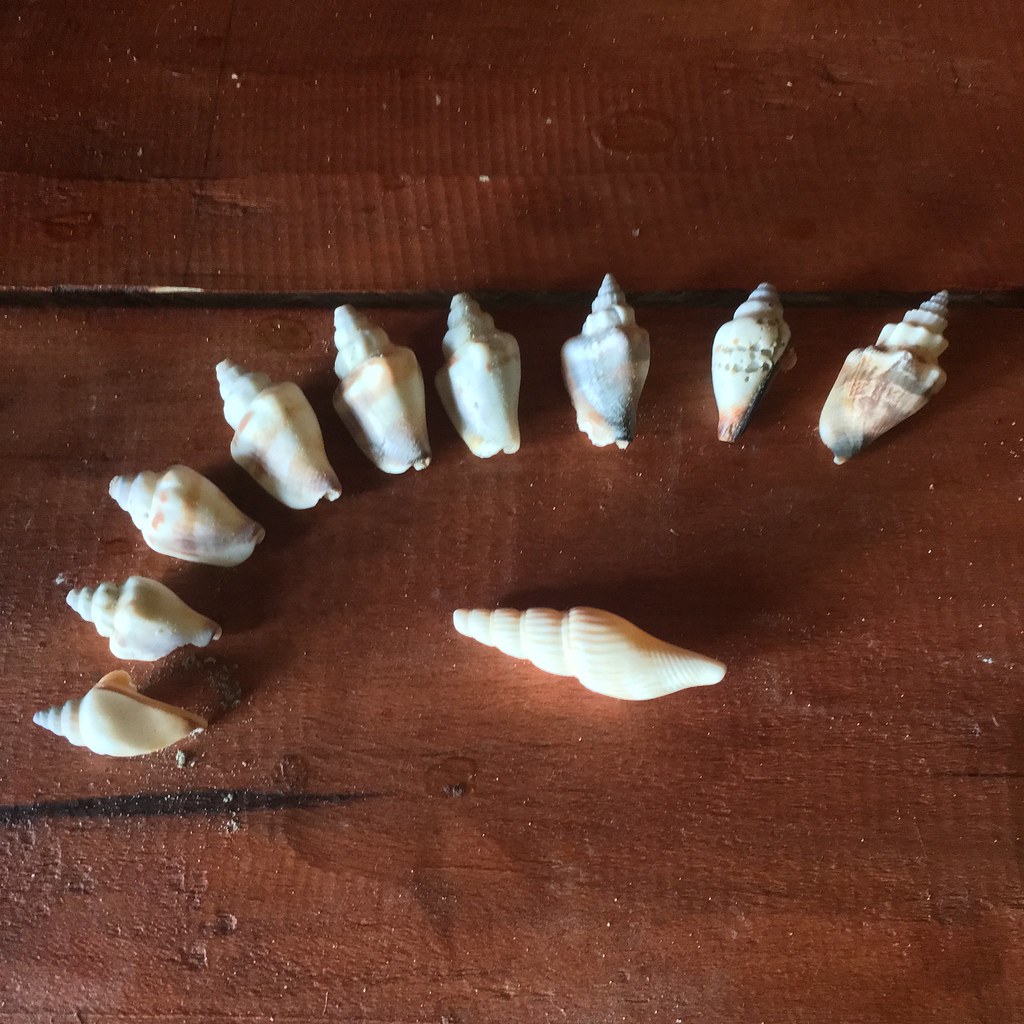This is a color photograph offering an overhead view of an arrangement of seashells on a dark brown wooden table composed of two horizontal planks. The upper plank covers about one-third of the image, while the lower plank spans the remaining two-thirds. On the bottom plank, nine small shells are strategically aligned in a curving formation that arches upward to the right. These shells exhibit a spiraling pointed top with curved, smooth bodies and are primarily white with occasional gray, brown, blue, and red hues. On the right side of this arched arrangement lies a slightly larger shell. Centered below this curving line is another entirely white shell, placed horizontally with its smooth end on the right and its spiraled end on the left. The wooden surface is dusty, lending a rustic touch to the composition.